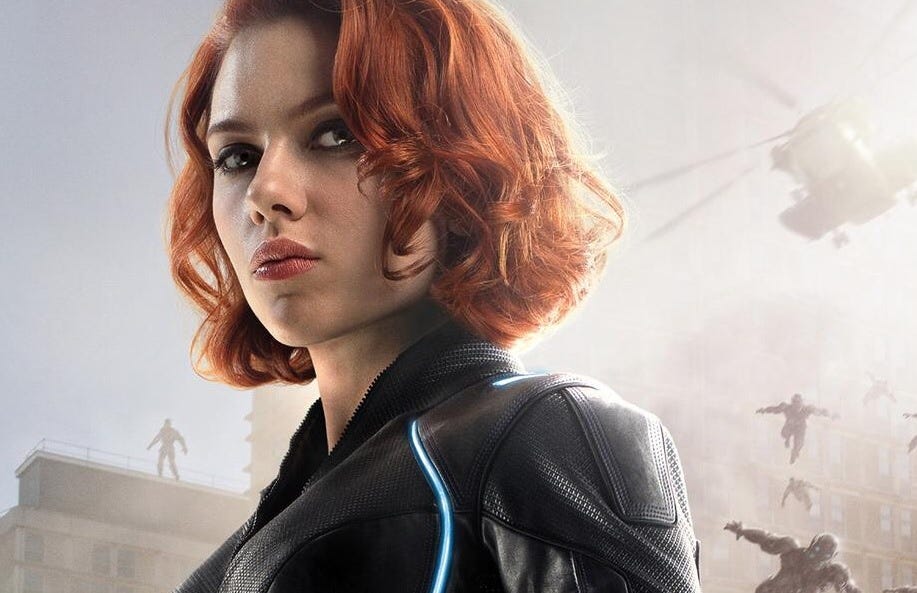In this striking close-up image, Scarlett Johansson, portraying her character from what appears to be a scene in the movie "Black Widow," is captured with a serious expression as she gazes directly into the camera. Her short, reddish hair, styled just above her shoulders with a slight curl, complements her light-colored eyes—likely green or hazel. Her makeup includes a bold red lipstick, enhancing the intense look on her face. She is dressed in a black leather jacket featuring a neon blue stripe running down the side.

The chaotic background contrasts sharply with her composed demeanor; a helicopter is prominently positioned in the top right corner, seemingly angling towards her. Beneath the helicopter, three figures—potentially appearing as aliens or men—are seen leaping through the air. The skyline behind Scarlett includes buildings shrouded in a smoky, foggy atmosphere, with one building on the left side where a lone figure stands on the rooftop. This amalgamation of elements suggests a dynamic, action-packed scene typical of a superhero movie, underscoring the intensity that Johansson's character exudes amidst the surrounding turmoil.